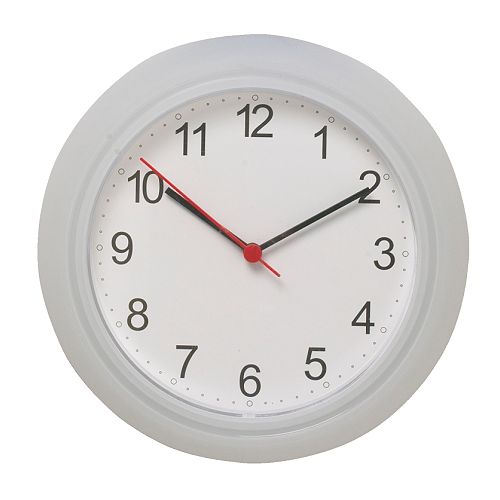A standard wall clock featuring a grayish-white outer band around its edge, which rises slightly to a thinner band of the same color positioned closer to the clock face. The face itself is a simple black-and-white design, displaying clear, plain Arabic numerals from 1 to 12. The clock has basic black hour and minute hands in the form of thin bars, complemented by a striking red second hand. Positioned around the edge at each numbered hour is a small circle, with tiny dots marking the individual five-minute increments between the numbers.